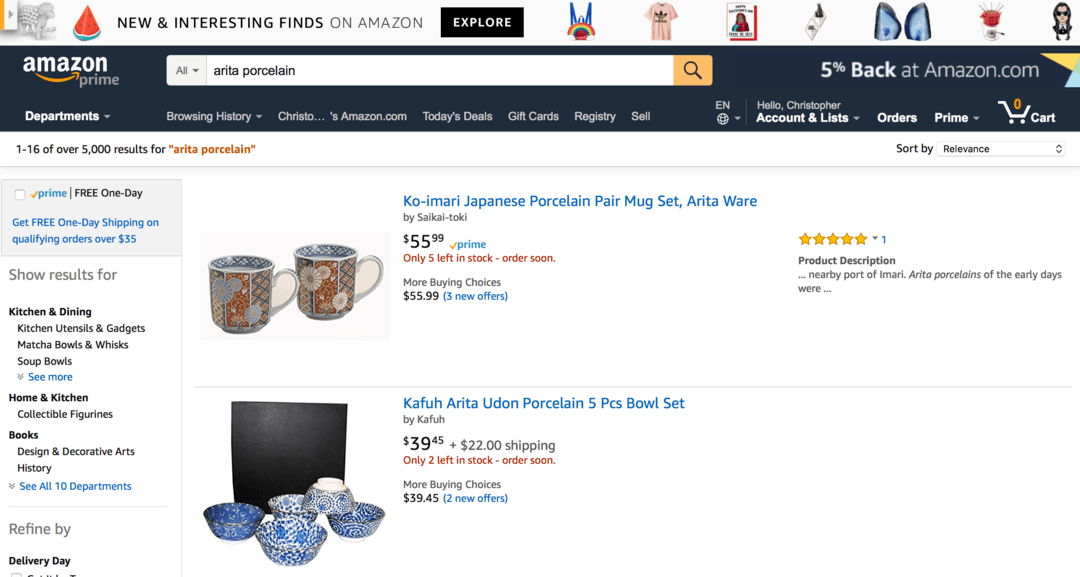The image has a light gray border at the top and prominently features an illustrated sheep alongside a slice of watermelon. A bold text overlay reads, "No Uninterested Finds on Amazon." Below the illustration, there is a black box containing the word "Explore." 

Underneath this black box, the Amazon logo is set against a black background. Within this black background is a search bar displaying the text "Arita Porcelain," accompanied by an orange box with a magnifying glass icon, indicating the search function.

Beneath the search bar, there is a listing for a product titled "Ko Amari Japanese Porcelain Pair Mug Set, Arita Ware, by Saki Toko," priced at $55.99 and available on Prime. The listing indicates that there are only five sets left in stock, urging customers to order soon. Additional buying options show the same price with three new offers available. The product boasts a perfect five-star rating from one review. The description highlights the historic significance of Arita Porcelain, referencing the port of Amari and early production days in the region.

Further down, the image also includes a mention of another product: the "Kafu Arita Udon Porcelain Five Piece Bowl Set."